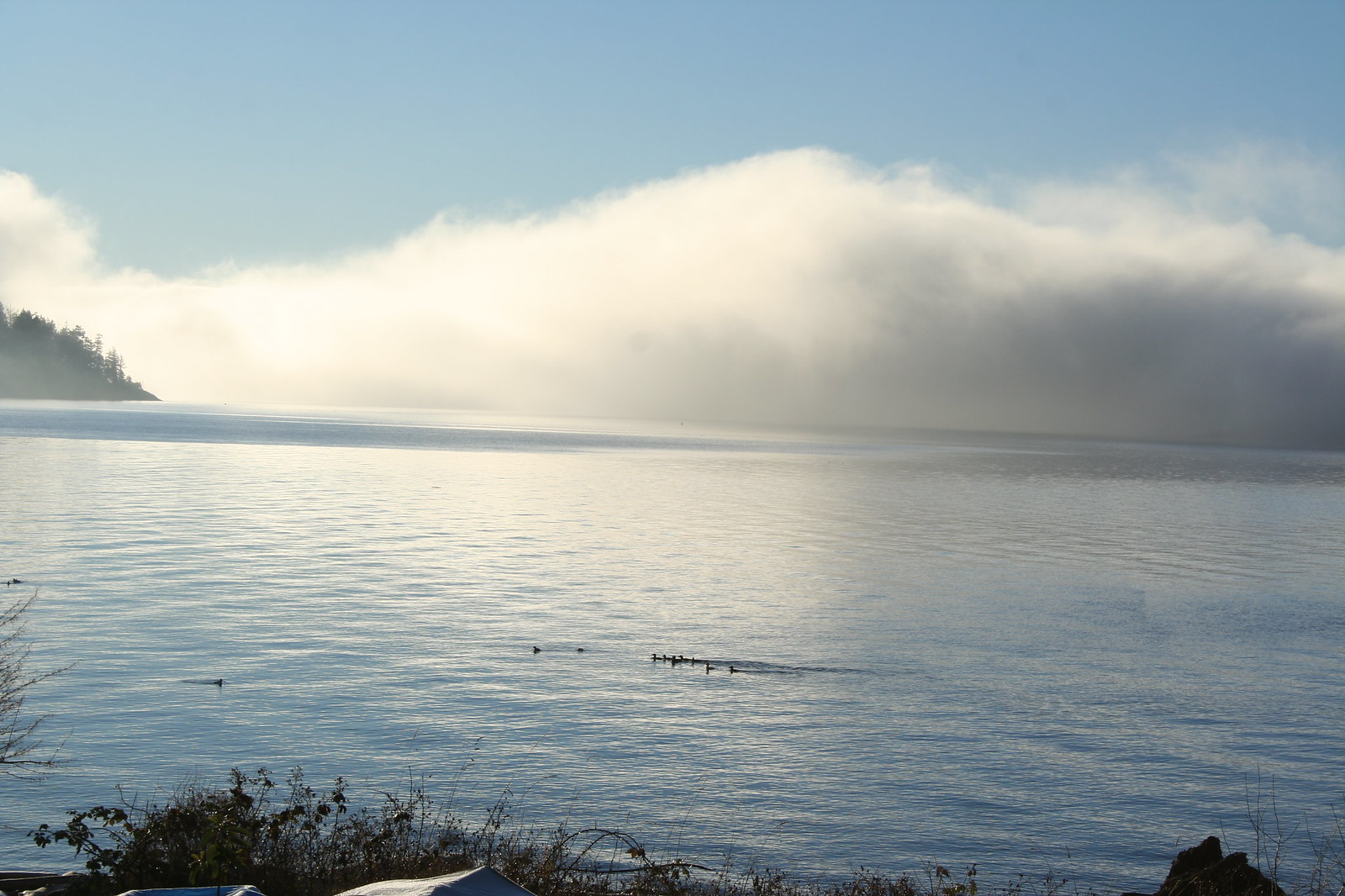This photograph captures a vast, serene lake stretching out to the horizon, with its calm, blue waters reflecting the soft light of a clear day. The sky above features a stunning contrast of a large white cloud that gradually darkens as it descends, set against a beautiful backdrop of blue sky. In the foreground, the shoreline is adorned with some grasses and shrubbery, while on the left side, a tree-covered hill gently rises. Scattered across the lake, a group of ducks can be seen swimming, their tiny silhouettes adding a touch of life to the tranquil scene. The peacefulness of the day is evident in the stillness of the water, which remains undisturbed by the wind, and the overall sense of calm and quiet is almost palpable.